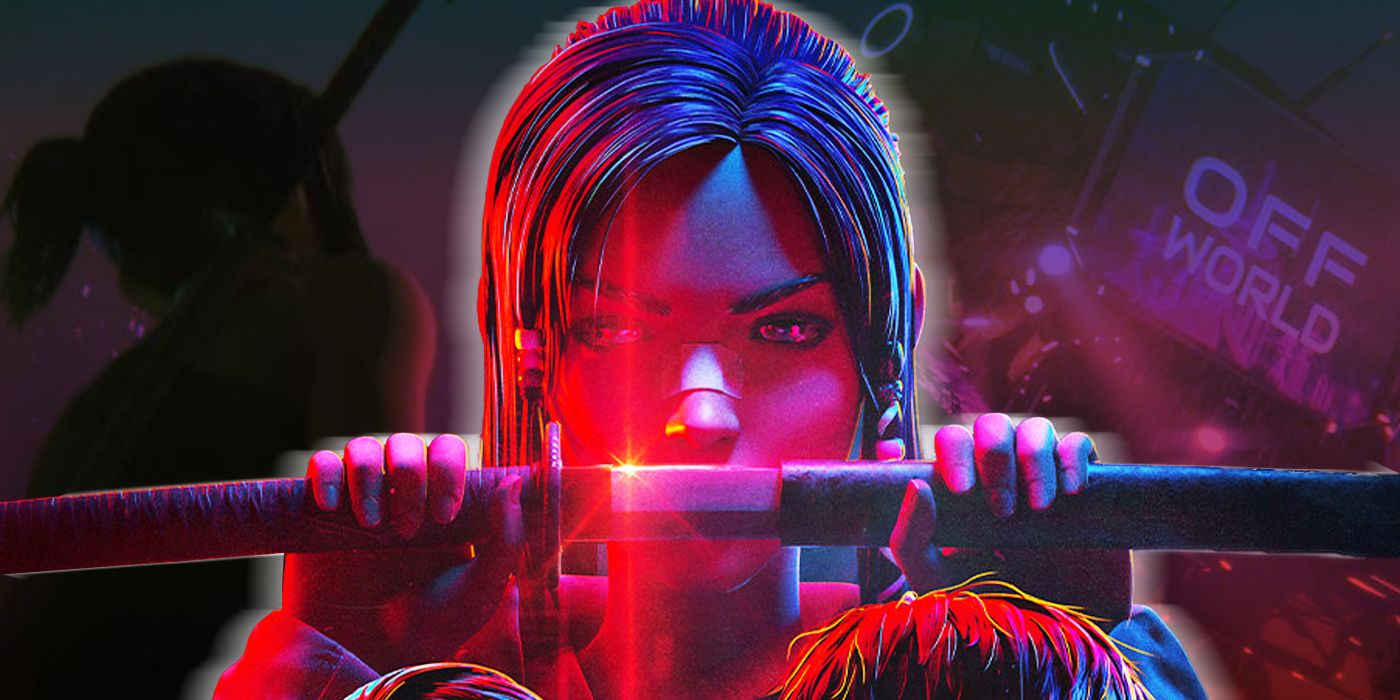In this animated image, likely from a video game, a female character with long, black hair stands at the center. Illuminated by red light, she holds a sword horizontally in front of her face, her left hand gripping the handle and her right hand on the sheath. The blade of the sword itself reflects a striking red glow. The character’s dark eye makeup and the red light accentuating her features and causing streaks in her hair add to her intense and focused appearance. The background features stark contrasts: the left side is shrouded in darkness with hints of a shadowy figure, while the right side is bathed in dark pink, purple, and red hues. In white text on the right, the words "Off World" are prominently displayed.